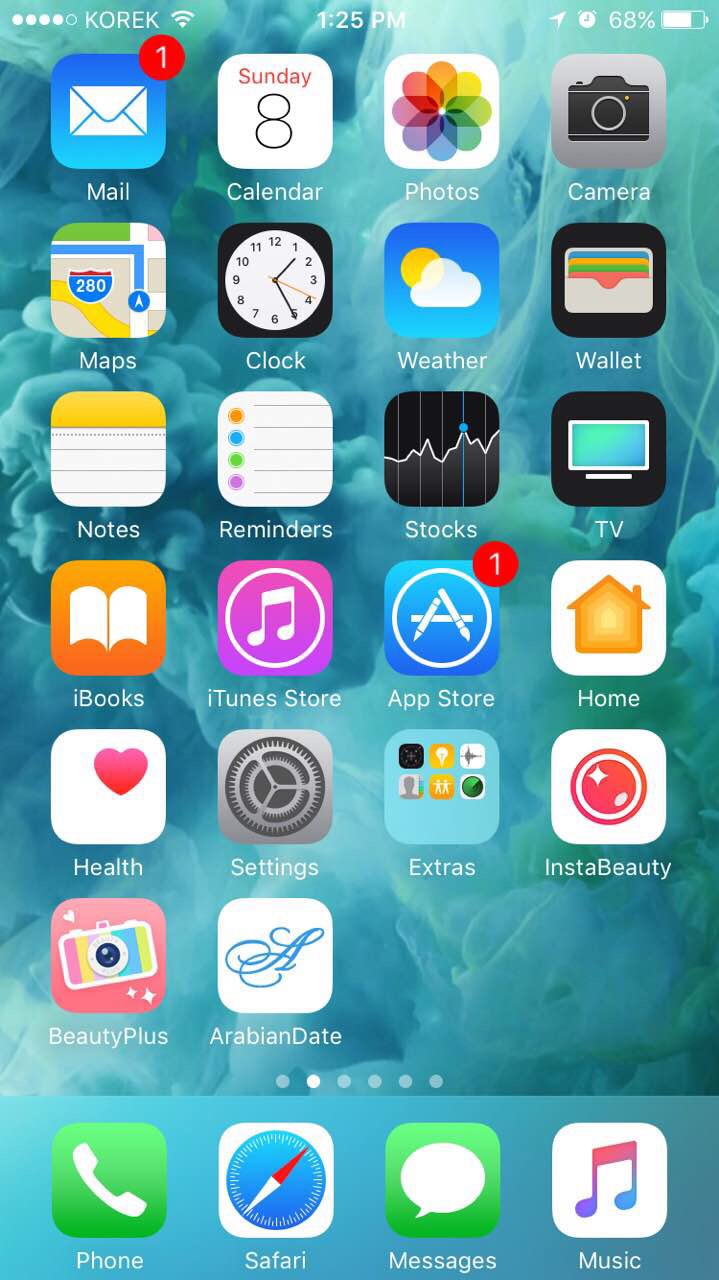This image is a detailed screenshot of a mobile phone's home screen. The wallpaper features an amorphous pattern composed of varying shades of blue. Displayed in the top-left corner is the label "Coric" in white text, accompanied by a series of five small circles—four filled and one empty—on its left side. To the right of "Coric" is the Wi-Fi symbol. Positioned in the center at the top of the screen is the time, shown as 1:25 p.m. On the top-right corner, the screen displays an alarm clock icon, a white arrow pointing to the upper right, and a battery icon indicating a 68% charge.

The home screen is populated with various app icons, organized into several rows. The visible apps include Mail, Calendar, Photos, Camera, Maps, Clock, Weather, Wallet, Notes, Reminders, Stocks, TV, iBooks, iTunes Store, App Store, Home, Health, Settings, Extras, InstaBeauty, Beauty Plus, and Arabian Date. Below these apps is a row of six dots, with the second dot from the left being white, indicating the current page, while the remaining dots are gray.

At the bottom of the screenshot is a dock with a light blue background, featuring four additional app icons: Phone, Safari, Messages, and Music. The display provides a comprehensive view of the user's organized and aesthetically pleasing mobile interface.